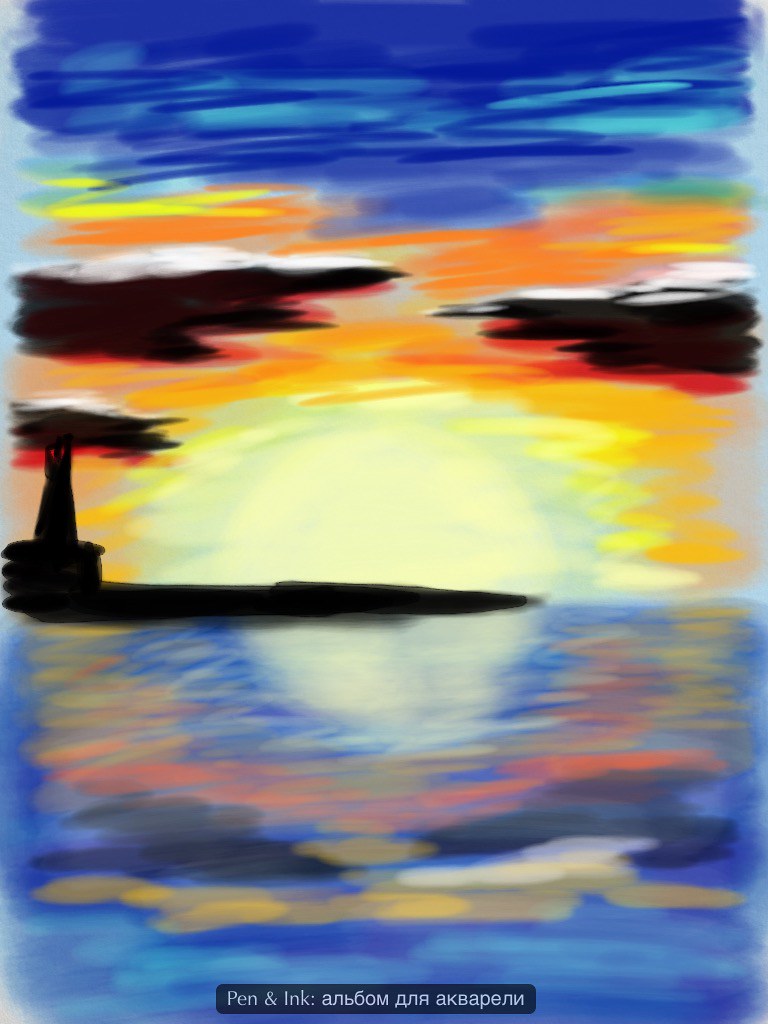This artwork appears to be a richly colored drawing, possibly created with paint, colored pencils, or markers. Predominantly featuring blue hues, it depicts a broad expanse of sky rendered in a gradient that transitions from dark blue to a light blue background towards the upper section. Interspersed within the dark blue sky are compelling streaks of yellow and orange, leading into a smaller section of white. Intriguingly, black accents emerge from both sides of the drawing, though they do not converge in the center. The focal point of the piece is a striking sunrise, consisting of a vibrant yellow and a lighter yellow semi-circle that represents the sun. Adjacent to and beneath the sunrise are subtle touches of black. Below this radiant scene lies a body of water, illustrated in blue and punctuated by reflections of the sunrise; streaks of yellow and orange shimmer across the water’s surface, mirroring the colors seen in the sky above.